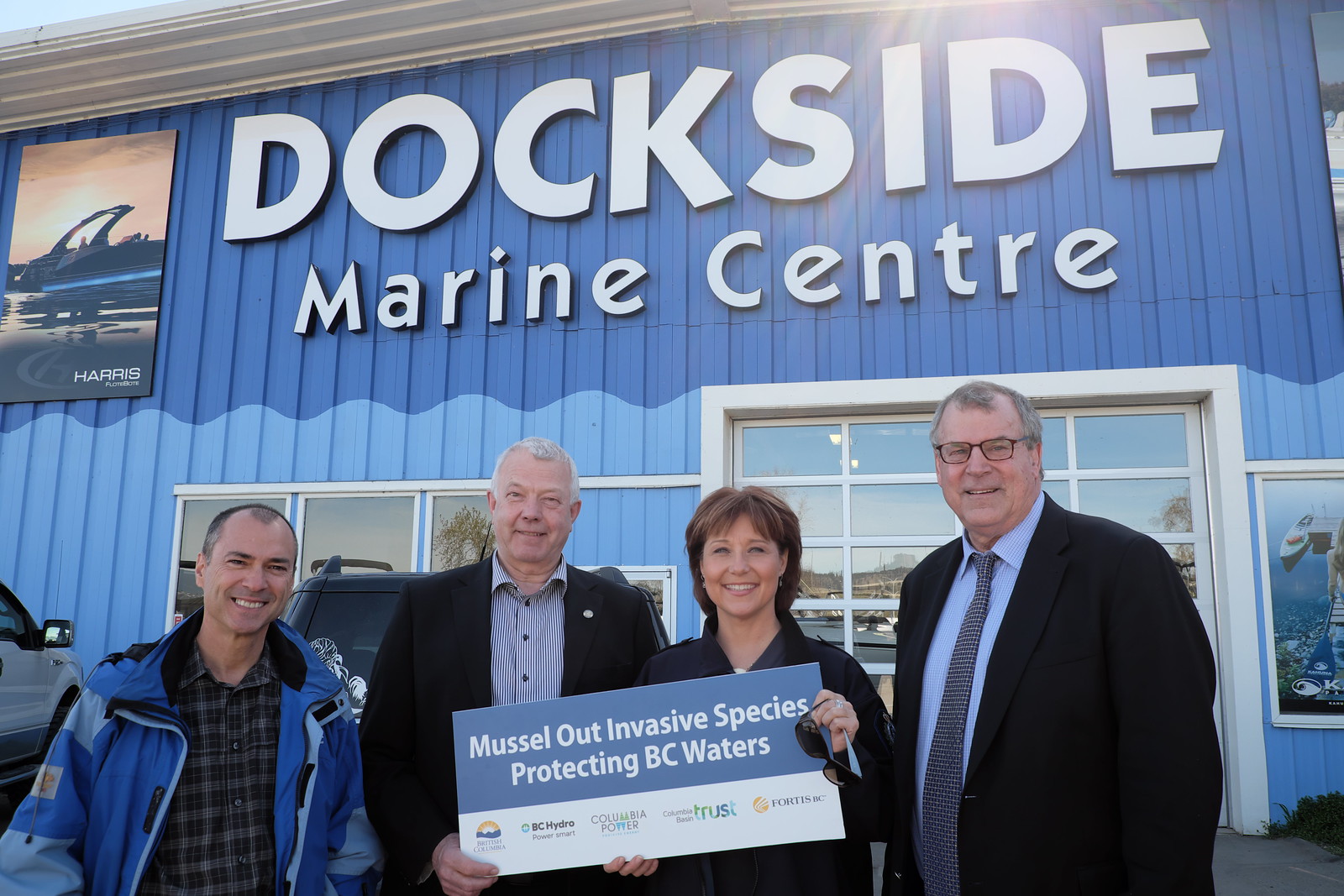In this full-color photograph taken outdoors during the daytime, four smiling individuals stand on an asphalt road in front of the Dockside Marine Centre, a blue metal building with big, bold white letters spelling out its name. The building features a detailed image of a boat in the upper left-hand corner, and it has several windows and an entryway visible from the front. The men and woman, who appear to be in their 40s and 50s, are dressed in coats and suits and are grouped with two men on the left, a woman in the middle right, and another man on the far right. The man and woman in the center are holding a sign that reads, "Muscle Out Invasive Species Protecting BC Waters," accompanied by five sponsor logos. The vivid colors in the image include blue, white, yellow, brown, black, gray, green, and various hues seen in the building, people's attire, and surroundings. This detailed and well-composed image captures a community effort to protect local waters from invasive species.